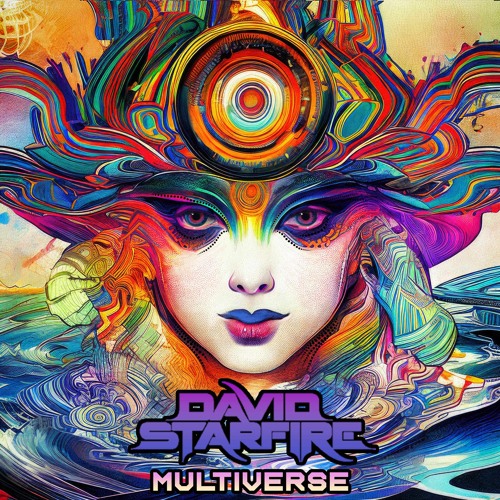The image is a vibrant and colorful square poster featuring a highly stylized woman's face. The woman has very white skin, brown eyes, and striking makeup with a blue upper lip and a red lower lip. Her eyes are adorned with dark purple eye shadow and surrounded by a blend of colors, including purple and red. The bridge of her nose transitions into yellow and blue hues, leading up to an elaborate, abstract headdress. This headdress consists of large concentric circles on the forehead, starting with a black outer border, transitioning to orange and blue, and culminating in an orange center. Bright streaks and ribbons of colors such as red, white, blue, light blue, purple, pink, and turquoise emanate from the headdress, creating a wavy, vibrant explosion of color around the woman's face.

Below the face, centered at the bottom of the poster, the name "David Starfire" is prominently displayed in futuristic text with a pink and purple gradient and a black outline. Underneath, in smaller, lighter pink and yellow gradient text with a black outline, the word "Multiverse" is written. The entire composition gives a sense of dynamic, multicolored energy, blending elements of anime and abstract art. The woman in the image is staring straight ahead, bringing focus and intensity to the overall design.